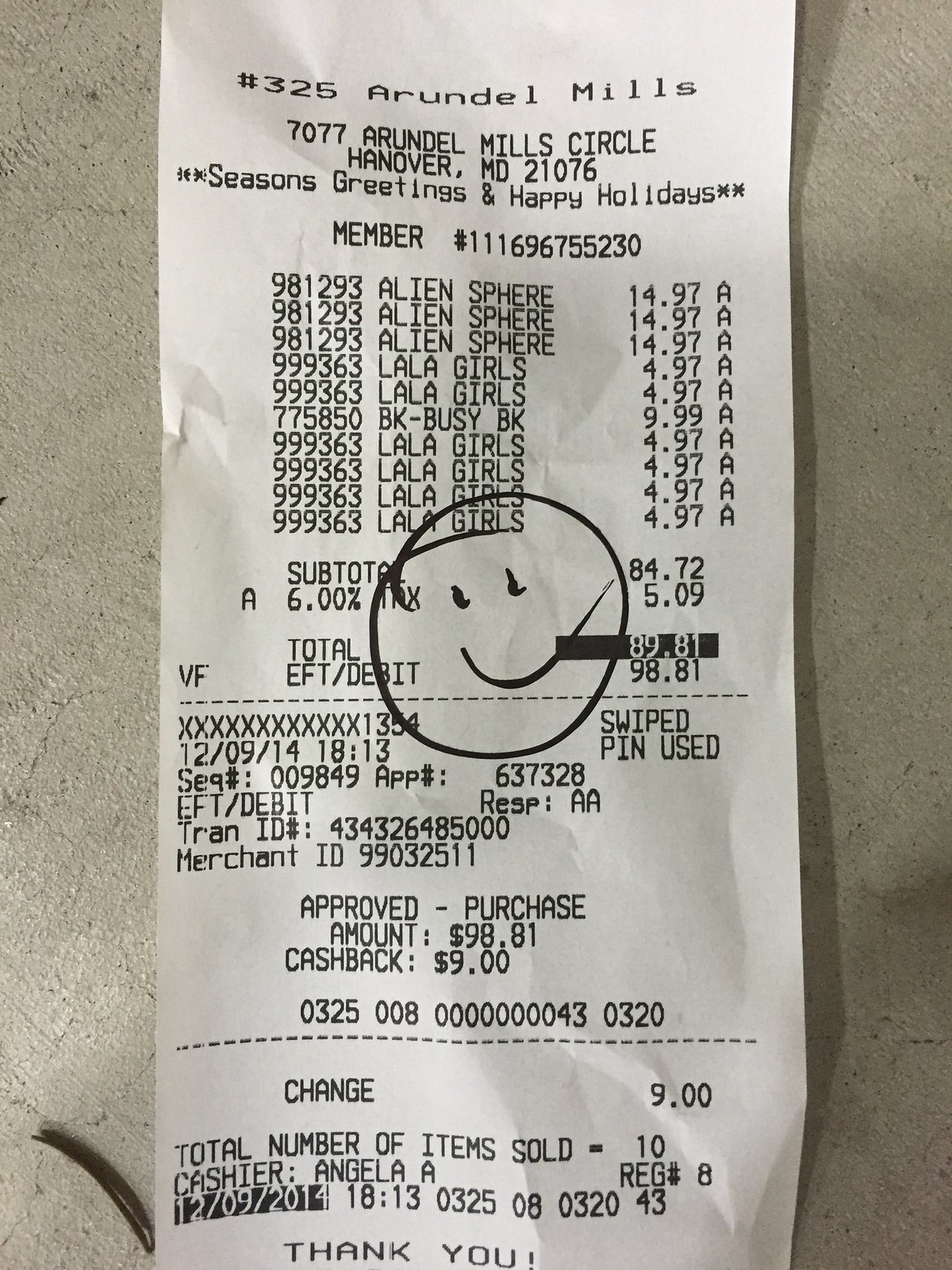A photograph of a receipt features a white background with black text. The receipt is resting on a somewhat dingy white surface. Prominently displayed towards the middle of the receipt, there is a black hand-drawn smiley face. At the top of the receipt, it reads "Number 325 ARUNDELMILLS," followed by the address "7077 ARUNDELMILLS Circle, Hanover, MD 21076." Below this, the phrases "Season's Greetings" and "Happy Holidays" are printed. The receipt lists various purchased items with individual prices, such as $14.97, $4.97, $9.99, and another item for $4.97, culminating in a total amount of $98.81. The purchase date is marked as December 9, 2014. At the bottom of the receipt, the printed message "Thank you" is visible.